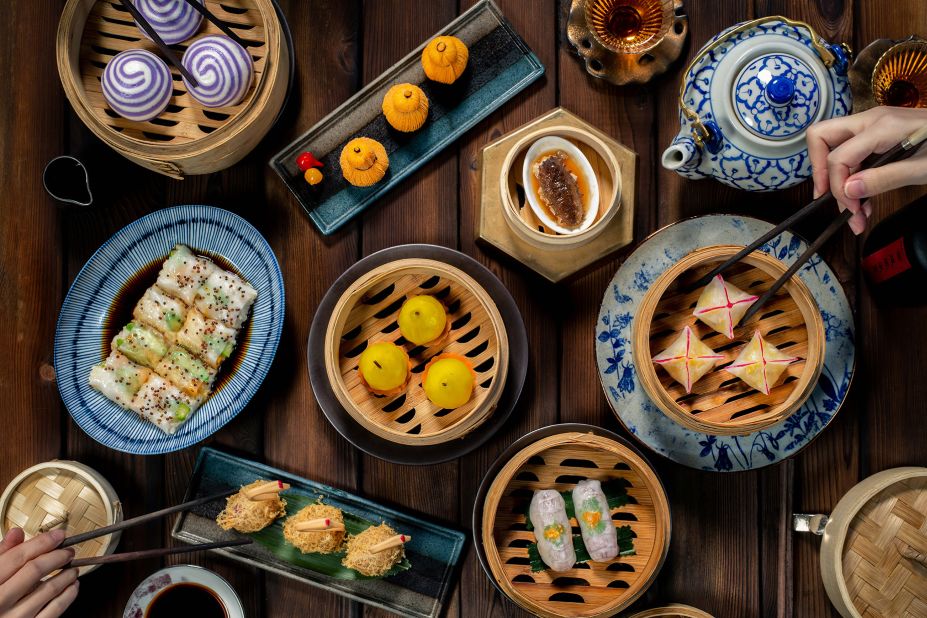From a straight-down perspective, this detailed indoor image showcases a wooden table with planks of varying shades of brown and black. Spread across the table are numerous dishes filled with a variety of Asian cuisine, primarily focusing on dumplings, potstickers, and wontons. Most of these delicacies are arranged within beige, naturally woven steaming baskets, although some items, including sushi and pastry-like dishes, are placed directly on the table. Complementing the colorful array of food, there are small bowls containing dipping sauces, and a distinctive blue and white teapot accompanied by matching teacups. The table settings also feature various plates, many of which are similarly blue and white. Two pairs of chopsticks being held by two individuals are seen reaching from the upper right and bottom left corners, capturing the dynamic interaction of the meal. This visually appealing scene highlights the rich and diverse selection of dim sum-style dishes being enjoyed communally.